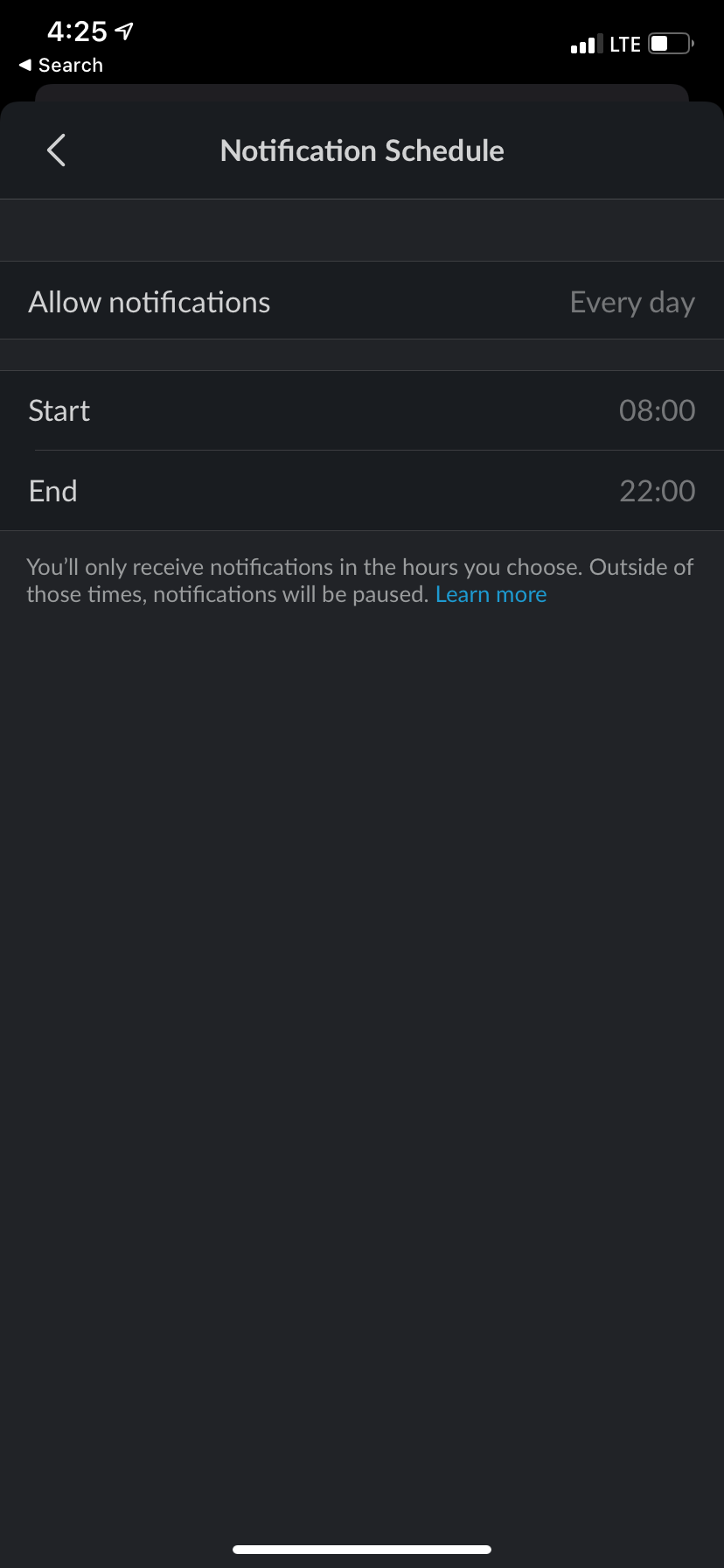The image is a screenshot taken from the screen of a mobile device, displaying a black background with white text and some gray elements. At the very top, it says "Notification Schedule." Below this, there is a faint gray bar, under which the text "Allow Notifications" is written in white. To the right side of this text, it says "Every day."

Below this, there is another light gray horizontal bar running the width of the screen. Beneath this bar, the text "Start" is written in white, and to its right, it indicates "0.8 hours." Similarly, further down, the text "End" is written in white, with "2200 hours" written to the right of it.

At the bottom of the image, there's additional white text stating, "You'll only receive notifications in the hours you choose. Outside of those times, notifications will be paused." Lastly, the text "Learn more" is written in blue.

This screen capture outlines the settings for configuring notification schedules, showing options to enable notifications during specified time frames only.